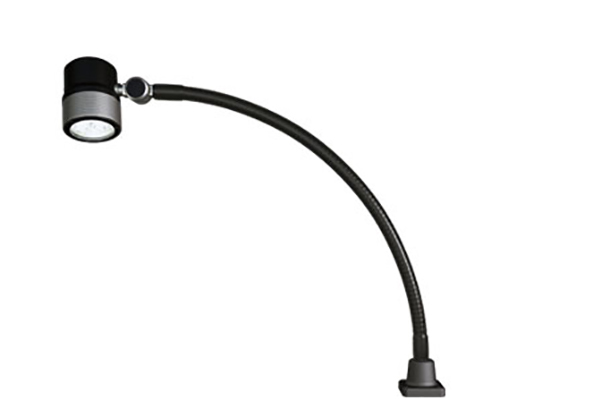This image depicts a bendable desk lamp set against a completely white background. The lamp features a small, metallic-looking black base positioned in the lower right corner. From this base, a flexible, pipe-like, black arm arches upwards to the left, demonstrating its adjustable nature. The arm connects to a metallic swivel joint at the top, which allows for directional adjustments of the lamp. The joint is characterized by a black button and silver accents. The lamp's head is cylindrical, resembling a small spotlight, with a distinctive design that includes a black top and a silver or gray bottom half. A white circular element is visible on the lamp's underside, likely indicating the light source. The overall design suggests versatility and adjustability, making it ideal for various lighting needs.